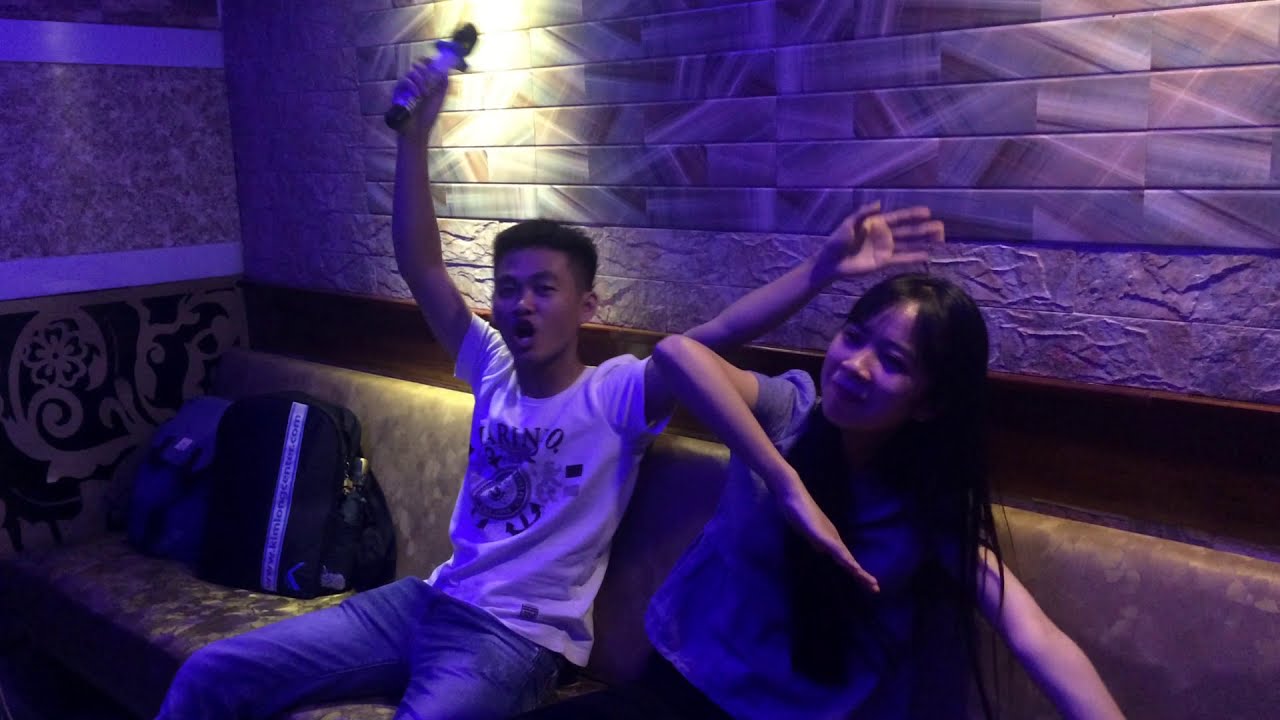In a dimly lit interior setting, which resembles a nightclub or karaoke room, two Asian teenagers are captured enjoying a lively moment. The hue of the image is painted with purplish lighting, adding to the festive atmosphere. Both are seated on what appears to be a long bench rather than a couch or a table. The young man, dressed in a white T-shirt with some partially legible text ("R," "I," and "N" visible) and blue jeans, is energetically extending his arms outward. He holds a microphone above his head, suggesting he might be singing or cheering. Next to him, the young woman with shoulder-length black hair supports herself on the bench with one arm while her other arm is outstretched in a playful karate chop gesture. She's smiling directly at the camera, adding to the vibe of enjoyment. In the background, a brick or concrete brick wall is partially illuminated by a light, highlighting the textures. Alongside them on the bench, there are two backpacks - one black and one light blue - hinting they might have brought some personal items. The overall scene vividly captures a moment of fun and celebration, suggesting they are reveling in the lively ambiance of a club or karaoke room.